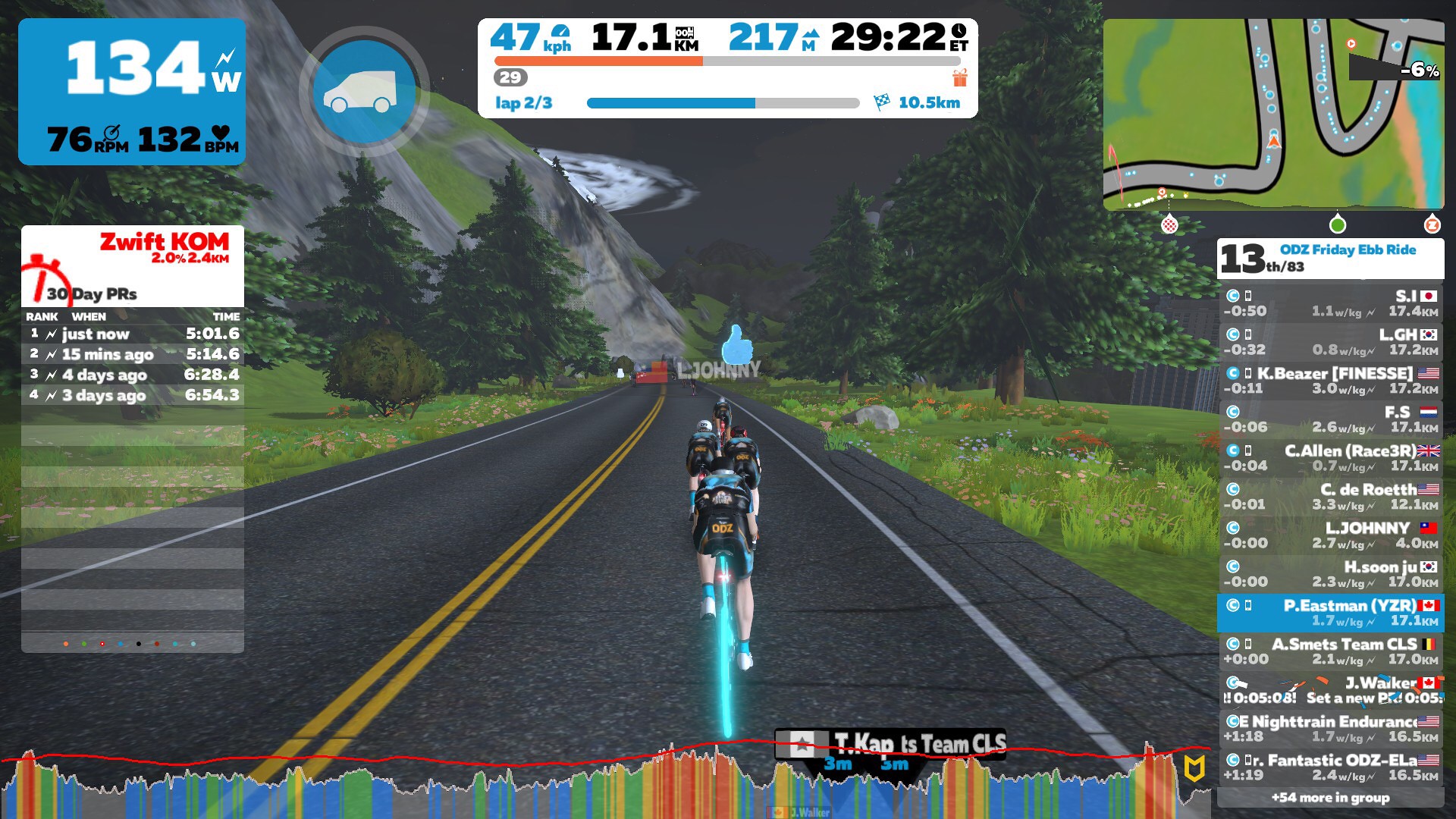In this detailed screenshot from a bicycle riding video game, we find ourselves behind a cyclist dressed in black, riding a lit-up blue bicycle on a regular highway with yellow lines in the center and white lines on the sides. The road is flanked by forests and mountains, leading downhill toward a water body with a big splashy puddle in the center of the cartoon-like scenery. 

On the right-hand side of the image, a leaderboard lists various players' names, their standings, and corresponding country flags. The title "13th Ooze Friday Eb Ride" is prominently displayed above the leaderboard. In the top right corner, a map of the route is shown, along with key statistics: 47 kilometers per hour (km/h), 17.1 kilometers (km), 217 meters (m) elevation, 29.22 elapsed time (ET), lap 2 out of 3, and 10.5 km completed in the lap.

To the left of these statistics, a smaller circular icon depicts a white truck on a blue background, accompanied by crucial metrics for the cyclist: 134 watts (W), 76 revolutions per minute (rpm), and 132 beats per hour (bph). Below, a chart from Wiftcom displays 30-day personal records with timestamps ranging from "just now" to "4 days ago." Additionally, a caption at the bottom right highlights "TCAP is Team CLS," and a thumbs-up icon with the name "Johnny" floats mid-screen, adding an interactive element to the user interface.